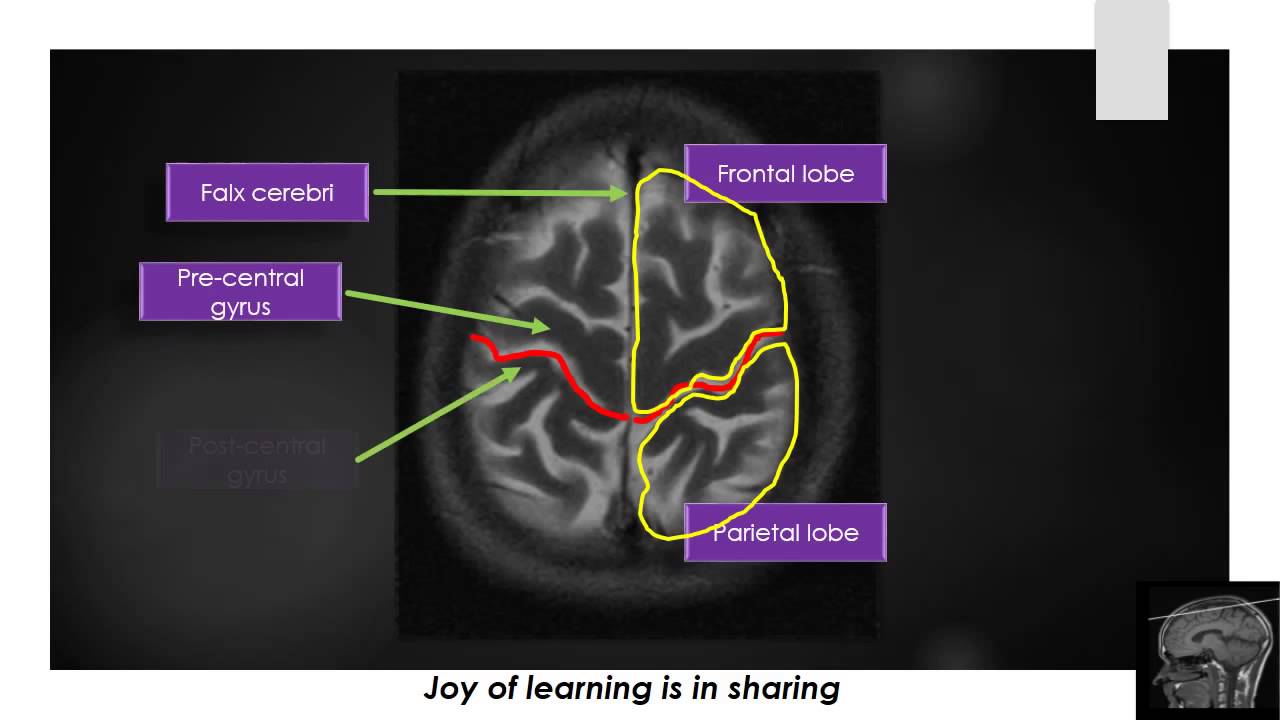The horizontal-rectangular image, predominantly black in background, displays a detailed scan of a human brain from a top-down view. Yellow and red lines trace various regions of the brain, connecting to purple boxes that label specific parts such as the "falx cerebri," "precentral gyrus," "frontal lobe," "parietal lobe," and "postcentral gyrus," with the postcentral gyrus label appearing slightly faded. Adding to the detailed annotations, green arrows are also employed to pinpoint these areas accurately. An additional inset at the lower right corner depicts a side view MRI of a person's skull, with a line illustrating the specific brain section shown in the main image. At the top right corner, there is a small, empty white box with no text. The image is framed within a white border, and along the bottom, in black text, it reads: "joy of learning is in sharing."